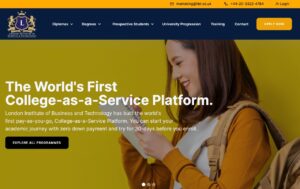A screenshot captures a section of a website showcasing an Asian student engaged with either a tablet or a ruled notebook against a vibrant yellow background. She is adorned in an orange overcoat, a white shirt, and carries a brown backpack slung over one shoulder. Her long brown hair frames her face, and she sports a touch of lipstick. Above her, a blue navigation bar featuring various website options and a contact phone number is visible, topped by a yellow bar. In the upper right-hand corner, there's a login option, though the low resolution limits clarity of further site details. Prominently displayed is the text "The world's first college as a service platform." At the bottom center of the image, three circles suggest auto-scrolling functionality, and a black button with indistinguishable text sits below them. The upper left corner is marked by an ornate letter 'L' embellished with intricate designs of horses and lions.